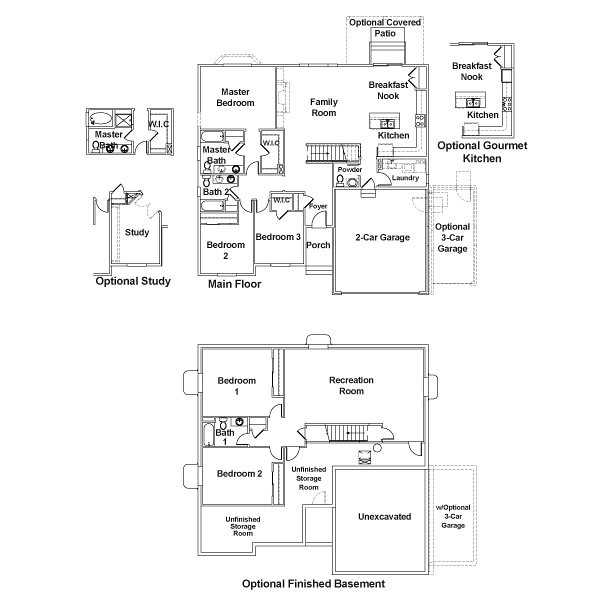The image depicts a detailed floor plan of a house, split into two sections: the main floor plan and an optional basement layout.

**Main Floor Plan:**
- **Upper Left Corner:** The master bedroom, paired with a master bathroom featuring a sink and a tub area. An optional study is situated below the master bathroom.
- **Lower Left Corner:** Two additional bedrooms labeled Bedroom 2 and Bedroom 3. Bedroom 3 has access to an adjacent porch.
- **Center:** The family room, accompanied by a breakfast nook and kitchen to its right. Above the breakfast nook lies an optional covered patio.
- **Below the Kitchen:** A functional laundry room and an adjacent possible bathroom.
- **Lower Right Corner:** A two-car garage with an optional extension for a third car.
- **Top Right Section:** The option for upgrading to a gourmet kitchen instead of the standard one.

**Optional Basement Layout:**
- Two additional bedrooms.
- A recreational room (rec room).
- A storage room.
- A three-car garage.
- An area marked as "unexcavated", indicating potential for further development.

This comprehensive floor plan offers a variety of optional features to suit different needs and preferences, presenting a versatile and customizable living space.